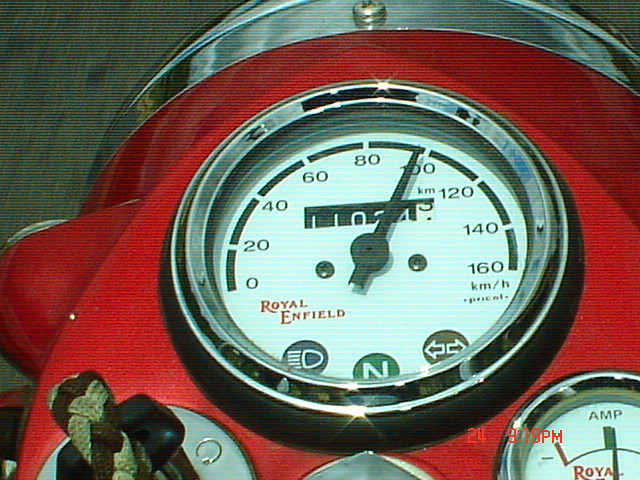The image captures a detailed view of a Royal Enfield motorcycle speedometer, prominently displaying a speed of 100 miles per hour. The circular speedometer integrates an odometer, tracking the total miles ridden. Adjacent indicators reveal whether high beams or turn signals are activated. A lower section of the speedometer is labeled "Royal," along with a notation "amp," presumably related to battery performance. A key adorned with a woven brown and cream rope is inserted in the ignition. The entire motorcycle dashboard is a striking red with numerous silver accents that reflect ambient light. The perspective suggests the photo was taken from a seat position, looking down. Below the dashboard, part of the roadway is visible, along with a left-side headlight and a designated footrest area. The reflective surfaces add a vivid, dynamic element to the composition.